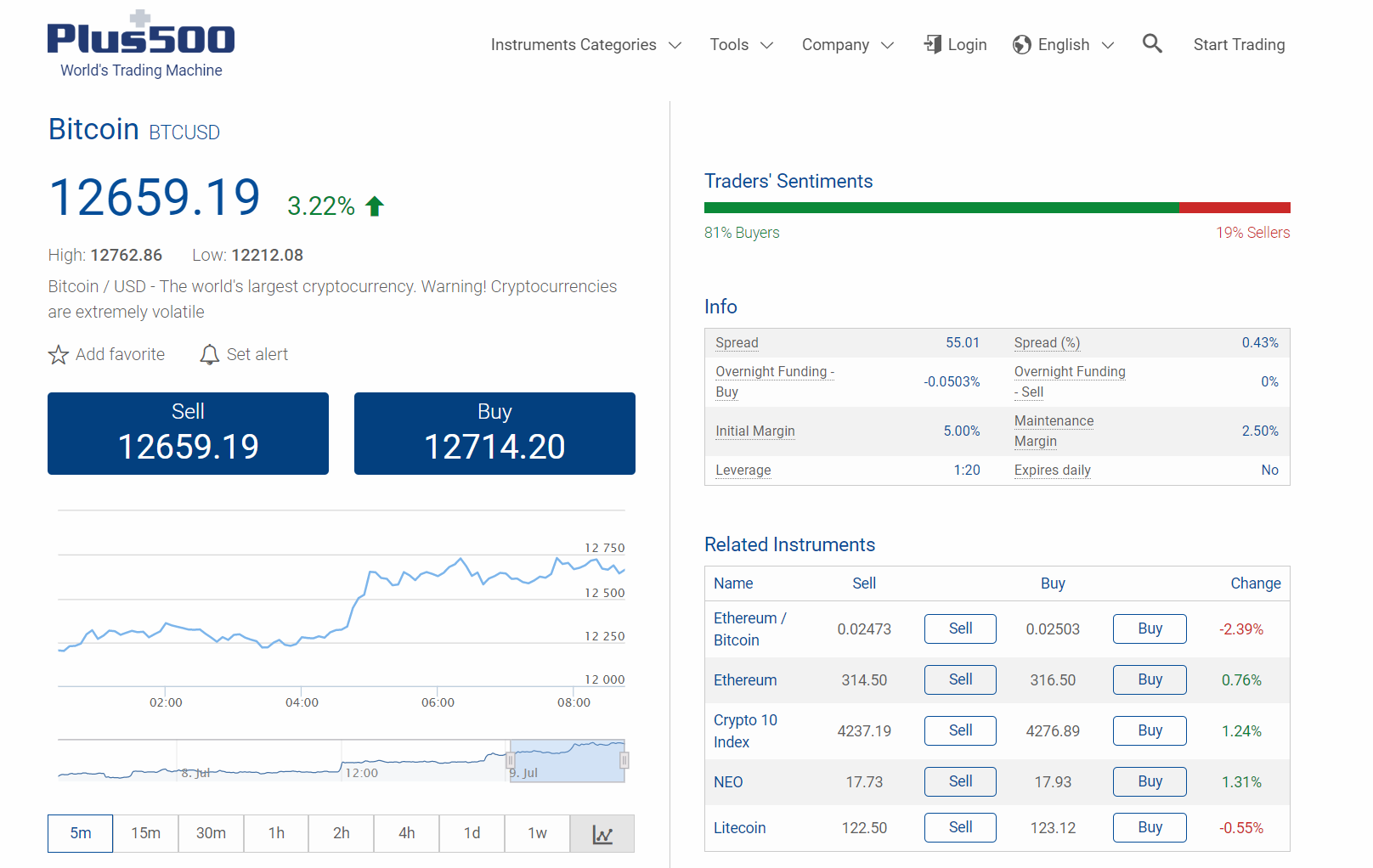A detailed, descriptive caption for the image:

"The image captures a computer screen displaying a line graph from the Plus500 world's trading platform, specifically focusing on Bitcoin (BTCUSD). The graph indicates upward movement, with two distinct trend lines: one showing a marked increase and another reflecting a more gradual ascent. The time frame selected for the graph is set to 5 minutes, although users have the option to view different intervals ranging from 15 and 30 minutes to 1 and 2 hours, as well as 4 hours, 1 day, and 1 week.

Prominently featured on the screen is a 'Traders Sentiments' section, illustrating that 81% of participants are buyers (highlighted in green), while 19% are sellers (marked in red). Below this, there is an informational segment detailing key parameters like spread, overnight funding, buy, initial margin, and leverage. Additional tabs provide further options such as 'related instruments,' showcasing various aspects necessary for a comprehensive trading experience."